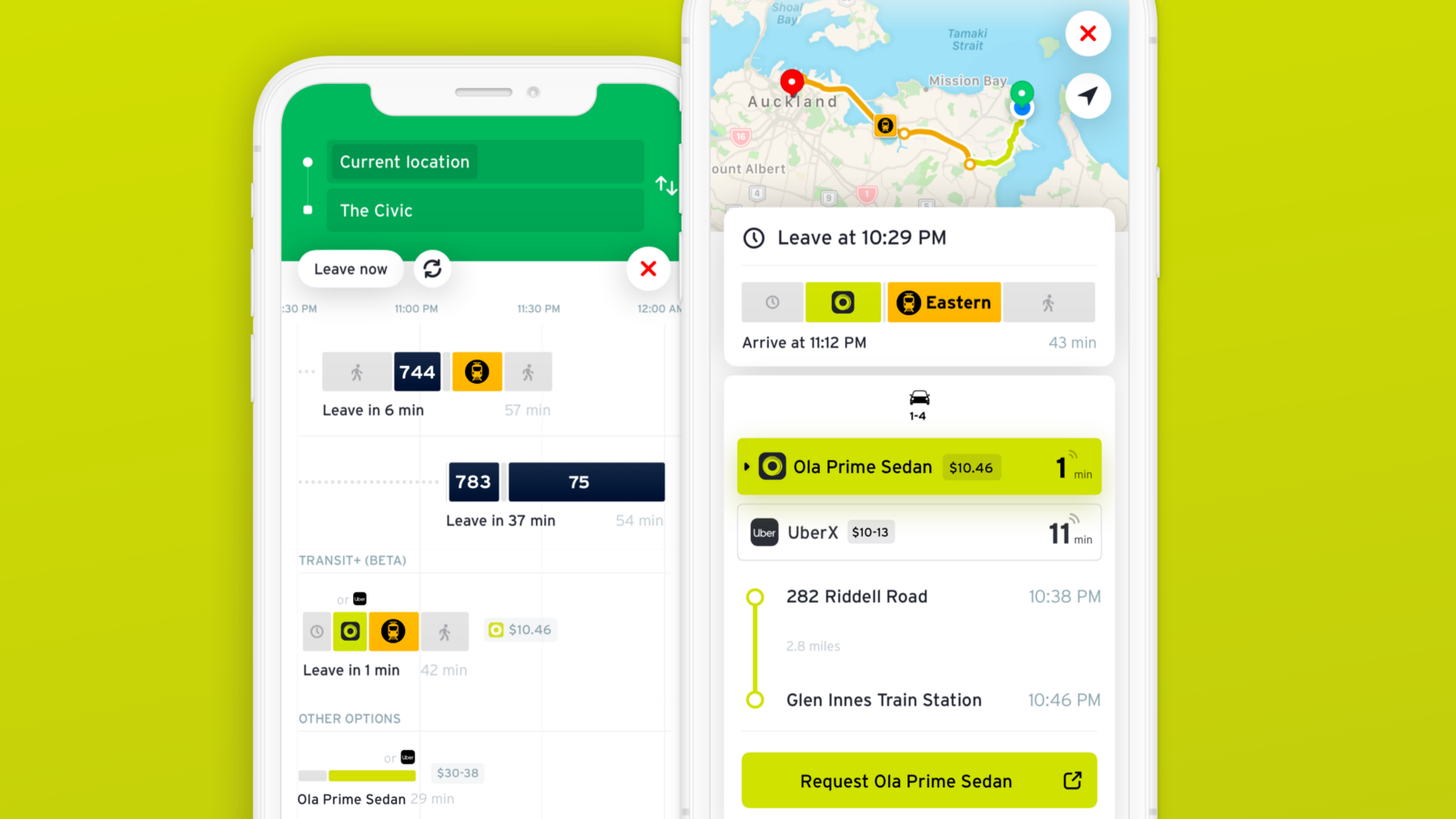The provided image showcases two vertically aligned screenshots of a navigation mobile app, set against a greenish-yellow rectangular background. The left screenshot features a user interface with a prominent green box at the top, designated for entering the current location and destination. Adjacent to these entries are arrows for swapping the origin and destination points. Below this is a setting to choose departure times, offering options for leaving immediately or at a later specified time. The interface includes multiple buttons for selecting different transportation modes such as walking, driving (gray button), public transit (black button, possibly a train icon), and various other black buttons for specific scheduling options like departing in 37 minutes. It also displays a calculated transit time below these options. 

The right screenshot displays a detailed map route, marked with a blue background indicating a body of water at the top. The route is illustrated winding across the geography, showing the path from the origin to the destination. Detailed trip information is provided at the bottom, including the departure time and transportation method. Notably, the details suggest an UberX sedan is the chosen mode of transport, with an arrival time either within a minute or an estimated travel time of 11 minutes to the destination.